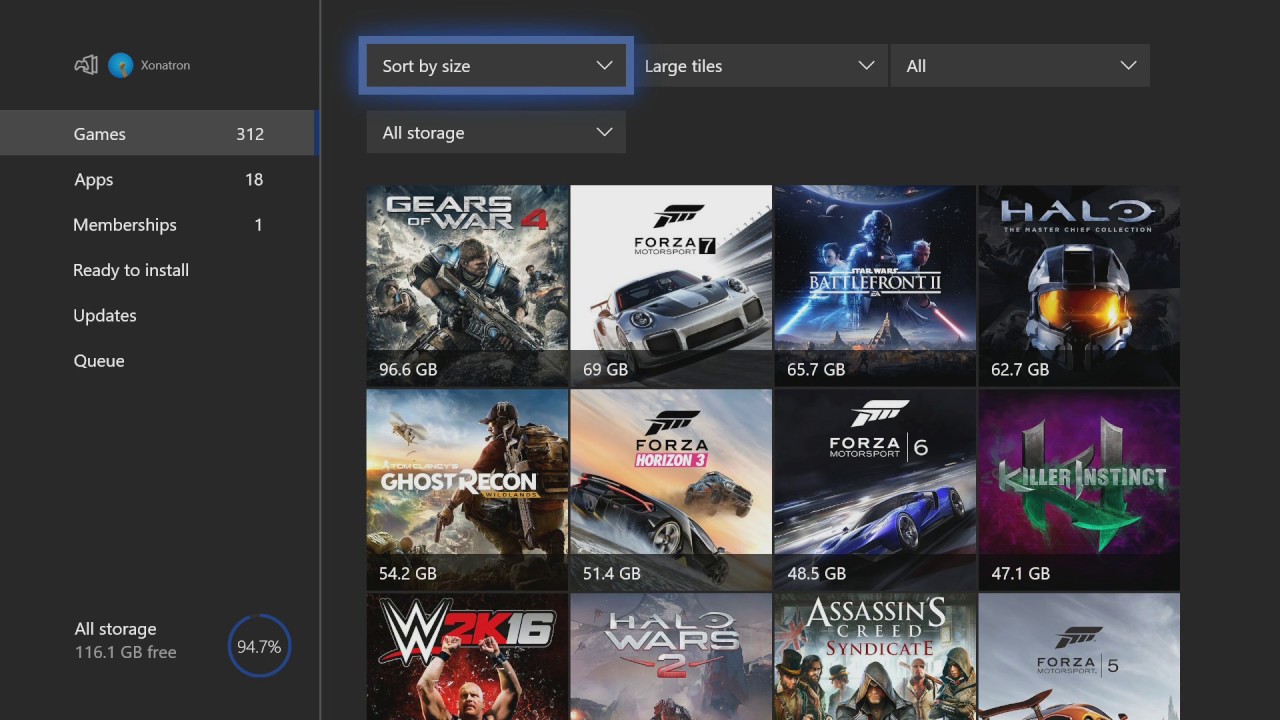A person is browsing their Xbox library, which is centrally displayed on the screen. In the top left corner, an icon featuring an Xbox console and controller is visible. To the right of this, there is a blue circular icon containing a character, though the details are hard to discern. Further to the right, the text "Xonatron" is displayed in light gray with the capital "X" followed by the lowercase letters.

The main menu is currently set to the "Games" category, indicated by the selection being highlighted in medium gray. Below this, the menu shows additional categories: "Apps" (18), "Memberships" (1), "Ready to Install," "Updates," and "Queue."

Toward the right side of the screen, a rectangular blue border highlights the "Sort by Size" option. Below this is a dropdown menu with options such as "Large Tiles," "All," and "All Storage."

Several game titles are listed underneath these menus, including:
1. Gears of War 4
2. Forza 7
3. Battlefront 2
4. Halo
5. Ghost Recon
6. Forza Horizon 3
7. Forza 6
8. Killer Instinct
9. WWE 2K16
10. Halo Wars 2
11. Assassin's Creed Syndicate
12. Forza 5

At the bottom left-hand side of the menu, "All Storage" is displayed in bold white text. Directly beneath, it indicates "116.1 GB free" in gray. To the right, a circle with a blue border—except for a split in the top left—shows "94.7%" in white text within the circle, signifying that the storage is 94.7% full.